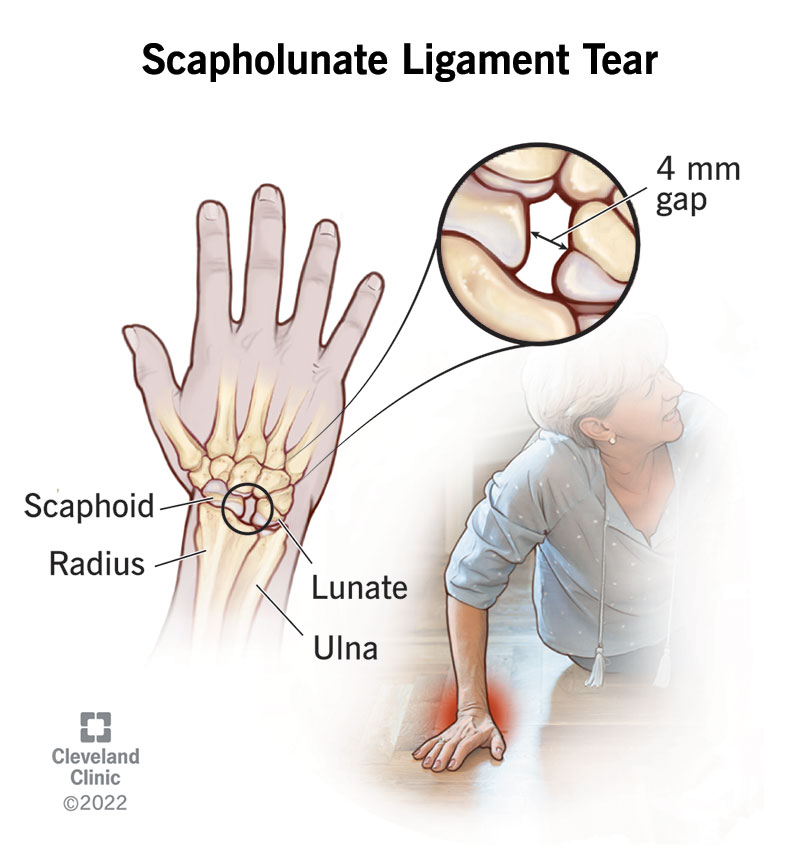This detailed annotated image from the Cleveland Clinic, copyrighted in 2022, illustrates a scapholunate ligament tear in the right hand. The main diagram on the left-hand side features a transparent view of the hand, allowing visualization of the underlying bones. Key bones are labeled, including the scaphoid bone at the wrist, the radius and ulna bones forming the forearm, and the lunate bone adjacent to the scaphoid. A notable detail is a zoomed-in circular inset showing a 4mm gap, indicative of the ligament tear, at the scapholunate junction. The bottom left-hand corner carries the Cleveland Clinic watermark and their square divided logo. Adding to the explanation, there is a background illustration of a woman who appears to have fallen, her hand pressing against the floor with a red radiating highlight around the wrist area to emphasize the pain and injury. The overall depiction effectively combines anatomical details with a visual representation of injury and discomfort.